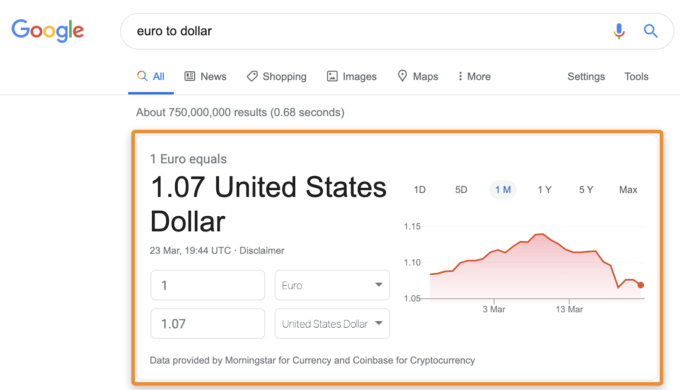This image shows a detailed currency conversion result from Google, displaying the exchange rate of 1 Euro to 1.07 United States Dollars. The data is stamped with the date "23rd of March, Universal Time," though the year is not visible. The conversion data is sourced from Morningstar and Coinbase, known for their financial and cryptocurrency services. The interface features drop-down menus that allow users to switch between different currencies or adjust the amount for conversion. A graph beneath the conversion rate illustrates the fluctuation of the Euro's value against the Dollar over the past month, showing a range between 1.05 and 1.15 USD. The graph's line is red, with a lightly shaded red area below it. The overall design of the page is minimalist, with a predominantly white background characteristic of Google's clean and straightforward layout.